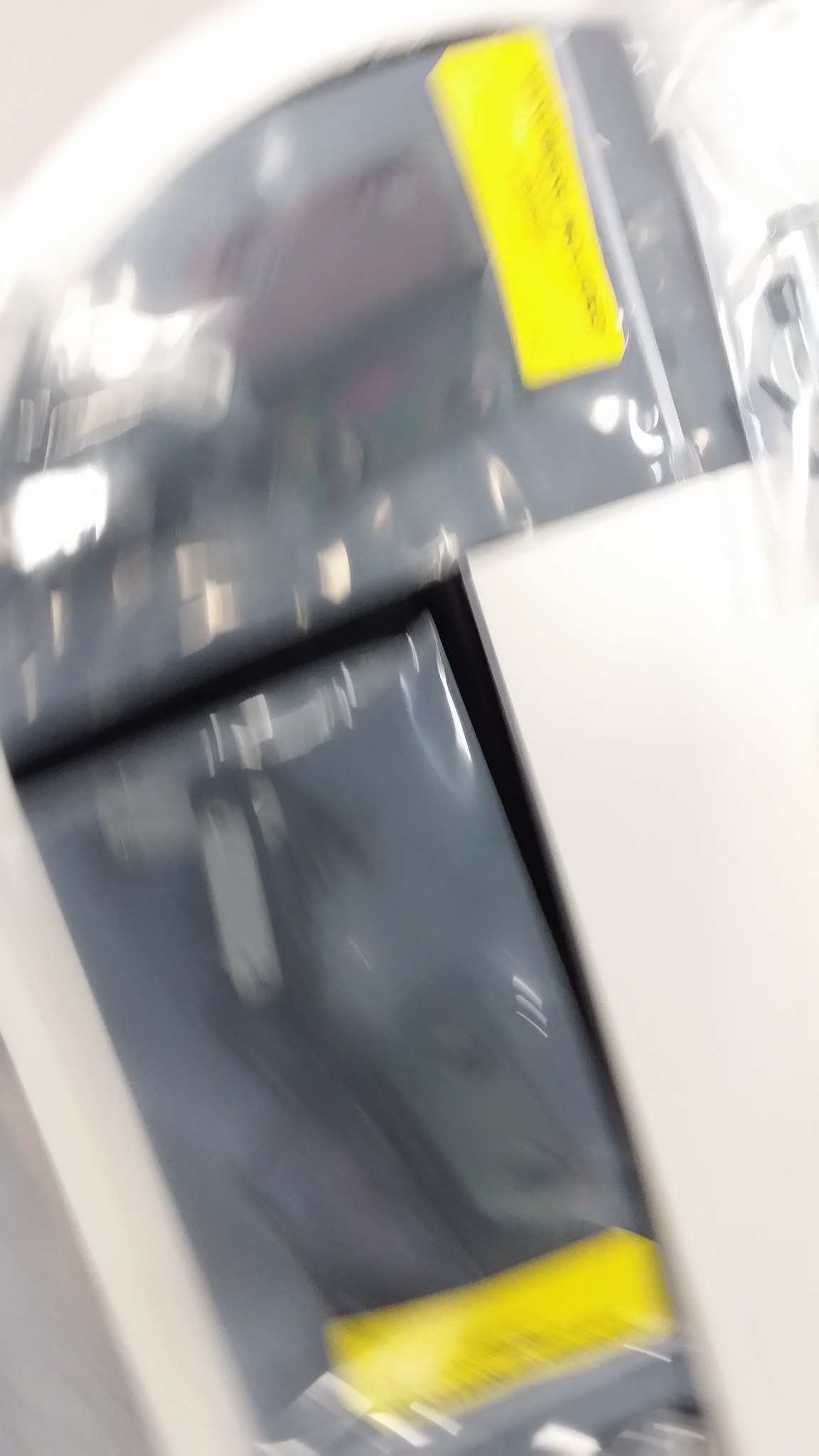The image depicts a sophisticated white container designed presumably to store and dispense plastic bags. The container features a semi-transparent plastic section, allowing for partial visibility of its contents. The top and bottom areas of the container each have a yellow tab, possibly for securing or opening the container. A more pronounced, rectangular segment of plastic extends downward from the top, with what appears to be a small tab protruding, potentially to facilitate opening. The outer shell of the container is made of sturdy white plastic, while the interior components seem to be constructed from a more flexible, lightweight plastic, making it easy to access the items inside. Despite the lack of definitive clarity on its precise function, the container's design suggests it is equipped to efficiently hold and dispense plastic bags.